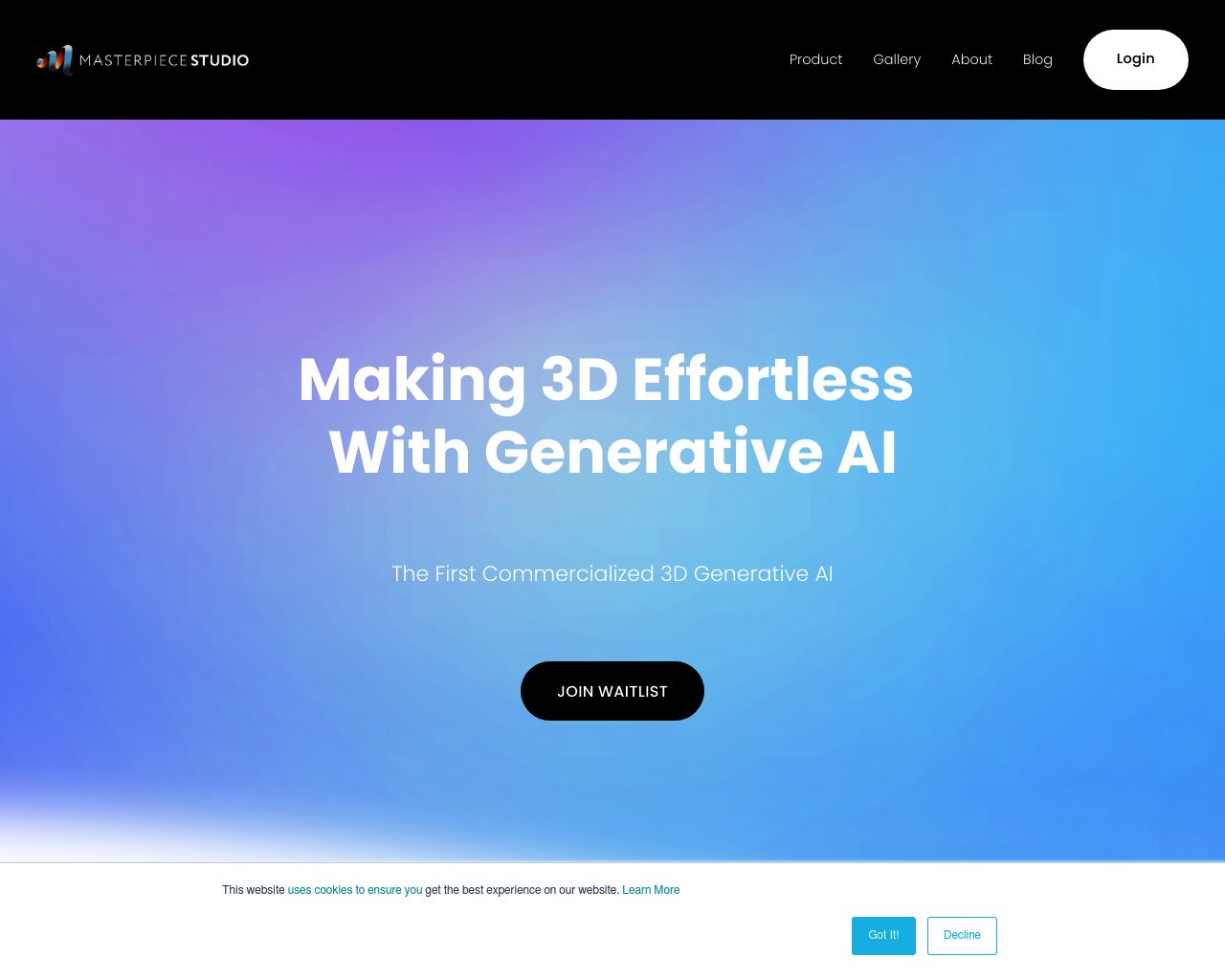The webpage designed by Masterpiece Studio is cleanly formatted for desktop view. The top of the page features a black banner with the Masterpiece Studio logo prominently displayed. The logo resembles three progressively larger, angular pillars connected by warm yellowish-red lights, resembling a Wi-Fi symbol.

Beneath the banner, there are five navigation buttons labeled: Product, Gallery, About, Blog, and Login. The main section of the page showcases a gradient background transitioning from purple to blue, and finally to a turquoise-ish dark blue. Overlaid on this gradient is the bold, white text: "Making 3D Effortless with Generative AI. The first commercial 3D generative AI. Join waitlist."

At the bottom of the page, cookie options allow users to manage their preferences with "Got it" and "Decline" buttons. Additionally, there's a note indicating, "This website uses cookies to ensure you get the best experience on our website. Learn more." Overall, the webpage embraces simplicity and clarity in its design, making it user-friendly and visually appealing.